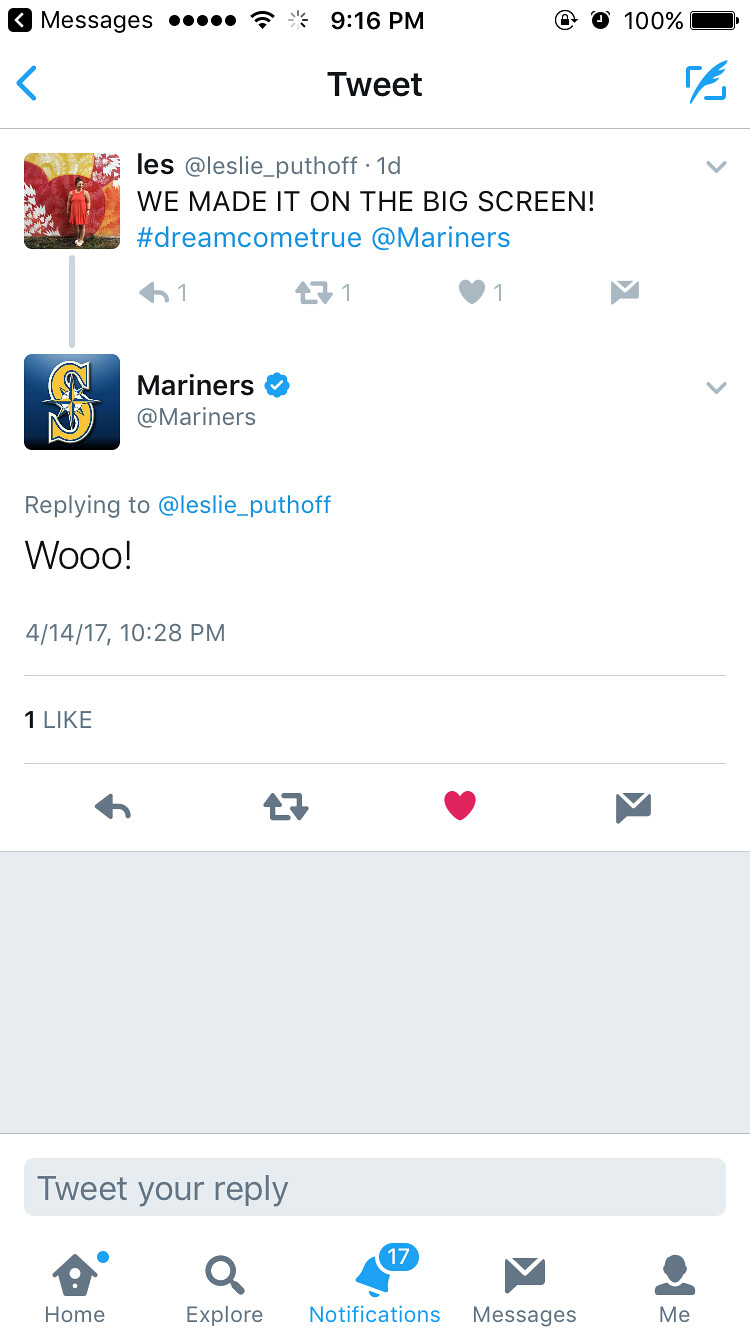The image depicts a screenshot from a mobile phone, showcasing a Twitter interaction between a user and the Seattle Mariners. The top of the screen displays standard mobile indicators, including the time (9:16 PM), signal strength, and a fully charged battery (100%). Below these, the Twitter app interface is visible. The header reads "Tweet," and beneath it, the tweet thread begins with a post by the user Les (username: @leslie_puthoff), made one day ago. Les excitedly shared, "WE MADE IT ON THE BIG SCREEN!!! #DreamComeTrue @Mariners." In response, the verified Mariners account (@Mariners) enthusiastically replied with, "Wooo!" This reply has garnered one like. The screenshot also reveals the Twitter bottom navigation bar, featuring icons for Home, Explore, Notifications (with 17 notifications), Messages, and the user's profile.